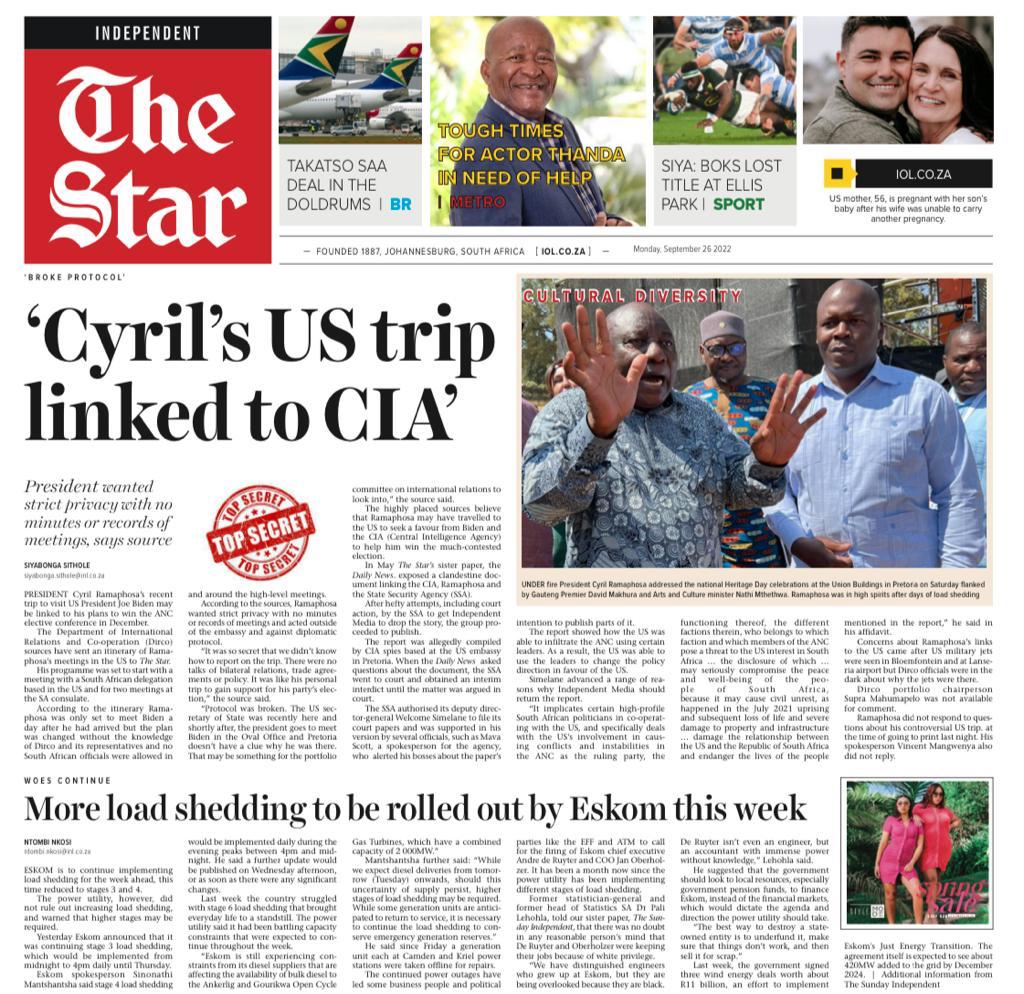Screenshot of an edition of "Independent The Star" newspaper featuring a detailed layout of news stories and images. The logo of the newspaper is prominently black and red. 

At the top of the page, there are four highlighted stories, each accompanied by a small image:
1. "Tecatso S.A.A Deal in the Doldrums" – Features an image of an airplane.
2. "Tough Times for Actor Thonda in Need of Help" – Accompanied by an image of a man.
3. "Sia. Box Loss. Title at Ellis Park, Sport" – Shows people playing a sport.
4. "U.S. Mother, 55, is Pregnant with Her Son's Baby After His Wife Was Unable to Carry Another Pregnancy" – Depicts a man and a woman.

The main story headline reads, "Searles U.S. Ship Linked to CIA," with a sub-heading on "Cultural Diversity." The accompanying photograph shows four black men dressed in blue with a woman barely visible in the background. This article is marked with a red "Top Secret" icon and extensive text.

Below the main story is another headline: "More Load Shedding to be Rolled out by ESCOM This Week," presented in a smaller format. Next to this, there's an image of two women dressed in pink, likely part of an advertisement for a "Spring Sale."

This newspaper page presents a diverse range of news topics and visual elements, capturing both local and international stories, alongside human interest pieces and advertisements.